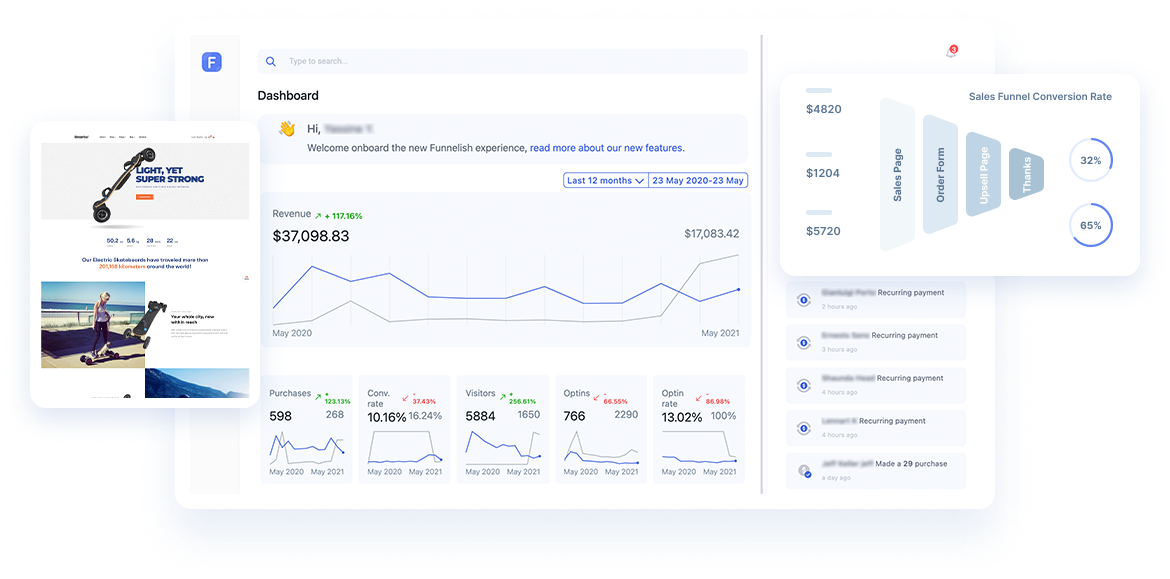The image showcases three distinct pages arranged side by side, with the left page appearing smaller in size compared to the other two. The central page is prominently displayed and resembles a dashboard from a financial portfolio webpage, featuring multiple line graphs accompanied by various numerical values. Highlighted on this page is a line graph with a significant figure of $37,098.83, suggesting an important financial metric. On the right, the final page mirrors the design of the central dashboard but focuses specifically on displaying a sales funnel conversion rate. The background across all pages is a clean, white color, contributing to a streamlined and professional aesthetic.